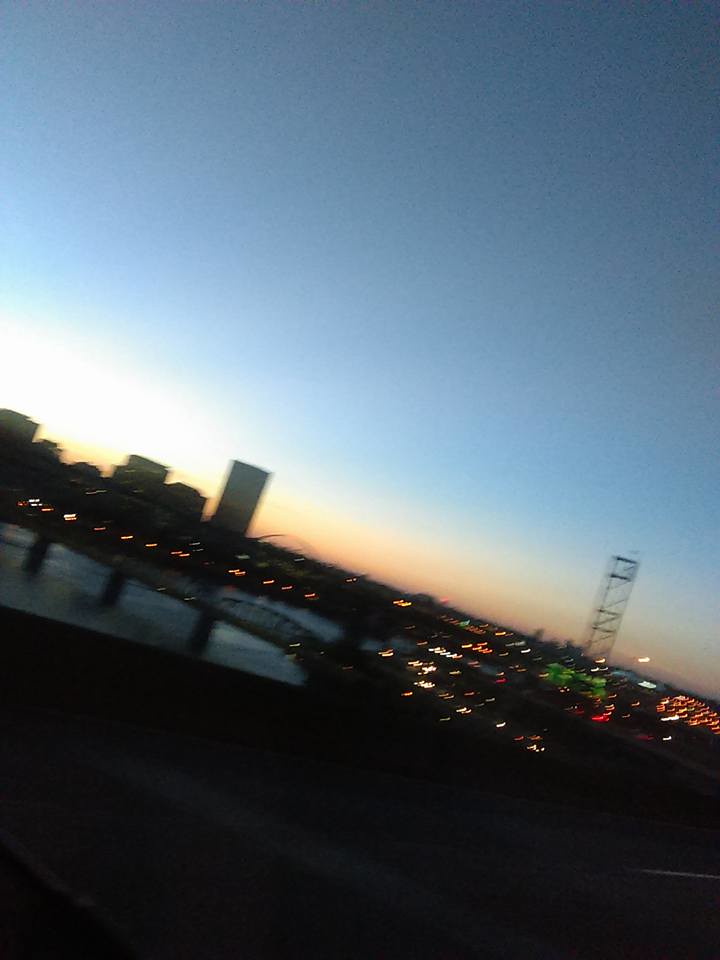An aerial photograph of a city skyline captured during the evening. The foreground is predominantly dark, lending a striking silhouette effect to the scene. To the left center of the image, a slightly tilted bridge spans across, adding an intriguing element to the composition. The city's skyline slopes gently downward towards the right, creating a dynamic visual flow. The upper portion of the image showcases the twilight sky, casting a serene backdrop to the city's bustling ambience. In the center, several buildings punctuate the skyline, their lights beginning to twinkle. Towards the right side of the image, the shimmering lights of vehicles and additional buildings hint at the city's vibrant nightlife.